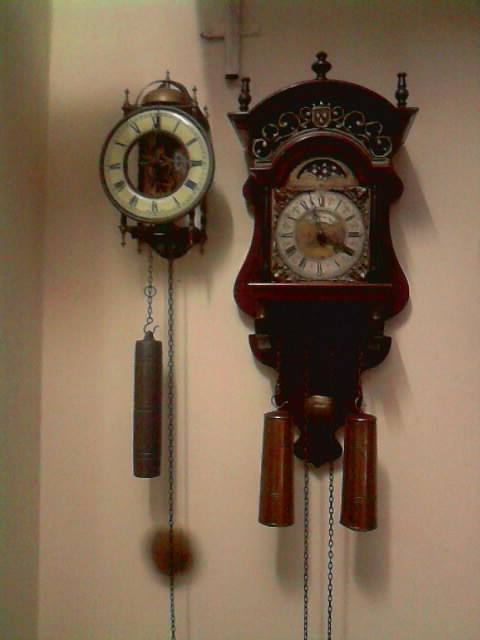This color photograph captures two ornate cuckoo clocks hanging side-by-side on a medium tan wall, which appears lighter due to the ambient lighting. Both clocks are intricate, with distinct characteristics and shared elements, such as Roman numeral dials and pendulums extending downward.

On the left is a smaller clock featuring a predominant pale yellow dial with Roman numerals. This clock stands out with its open back, showcasing a brass domed bell at the top. Another unique feature is its heavy-looking brass pendulum, accompanied by a long, delicate chain. The clock structure is minimalistic compared to its counterpart, focusing more on the dial rather than an ornate enclosure.

The larger clock on the right has a more architectural feel, housed in dark mahogany-like carved wood that rounds into an ornate shape. The slightly smaller white dial with Roman numerals is set within a square brown inlay. Above the clock face, a decorative, crown-like structure adds to its grand appearance. At the bottom, two large wooden pendulums and a chain hang down, emphasizing the clock's complexity. This clock is noted for its dual weights, which are more prominent than the single weight on the left clock.

The detailed shadows on the wall behind the clocks suggest lighting from above, casting an intriguing dimension to the scene, enhancing the appearance of these beautifully crafted timepieces.